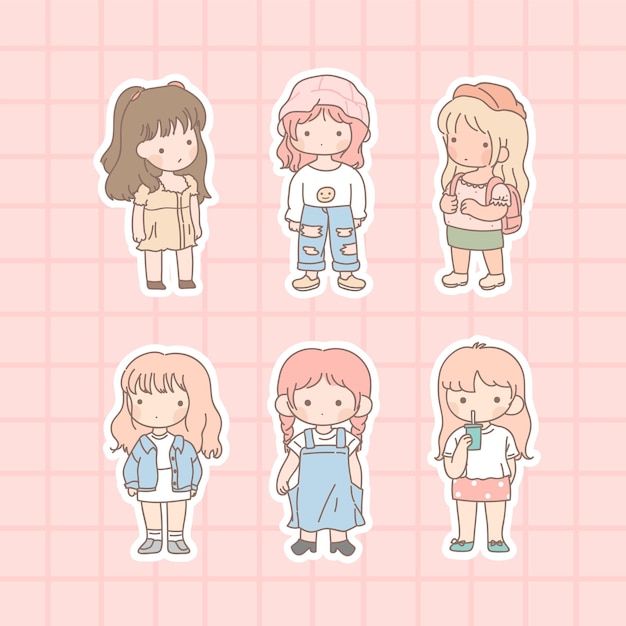The image is a playful scene featuring six cartoon stickers of little girls, all outlined in white, set against a backdrop of light pink squares and darker pink borders forming a grid pattern. Each sticker showcases a different girl with distinct characteristics and outfits. In the top row, the first girl has long brown hair and wears a pale yellow dress. The middle girl sports a pink bucket hat, ripped jeans, and a white long-sleeve t-shirt. The third girl has long blonde hair, an orange cap, a pink frilly shirt, a dark pink backpack, and a green skirt. On the bottom row, the first girl, with light red hair, wears a blue jacket over a white shirt and white skirt. The middle girl has red pigtails, a white t-shirt, and a blue denim dress. The last girl on the right has light red or pink hair and is sipping from a drink with a straw, dressed in a white t-shirt and a pink skirt. All the girls have simple facial expressions with two eyes, no noses, and small dot-like mouths, giving them an inquisitive, neutral look.